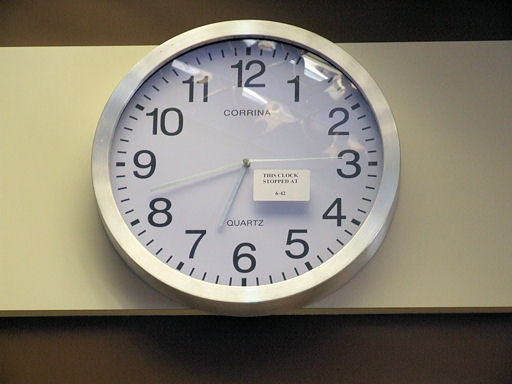This photograph captures a circular clock prominently displayed on a section of the wall. The wall itself is brown, providing a stark contrast to the off-white rectangular block affixed to it. The clock, featuring a sleek silver metal border, rests centrally on this white block, suggesting it might be part of an exhibition or a curated display. The clock face is white, with clearly defined black numerals and a straightforward, functional design. Notably, atop the clock's glass cover, there's a white sticker with black text that reads, "This clock stopped at 6:42," adding a narrative and sense of curiosity to the scene.